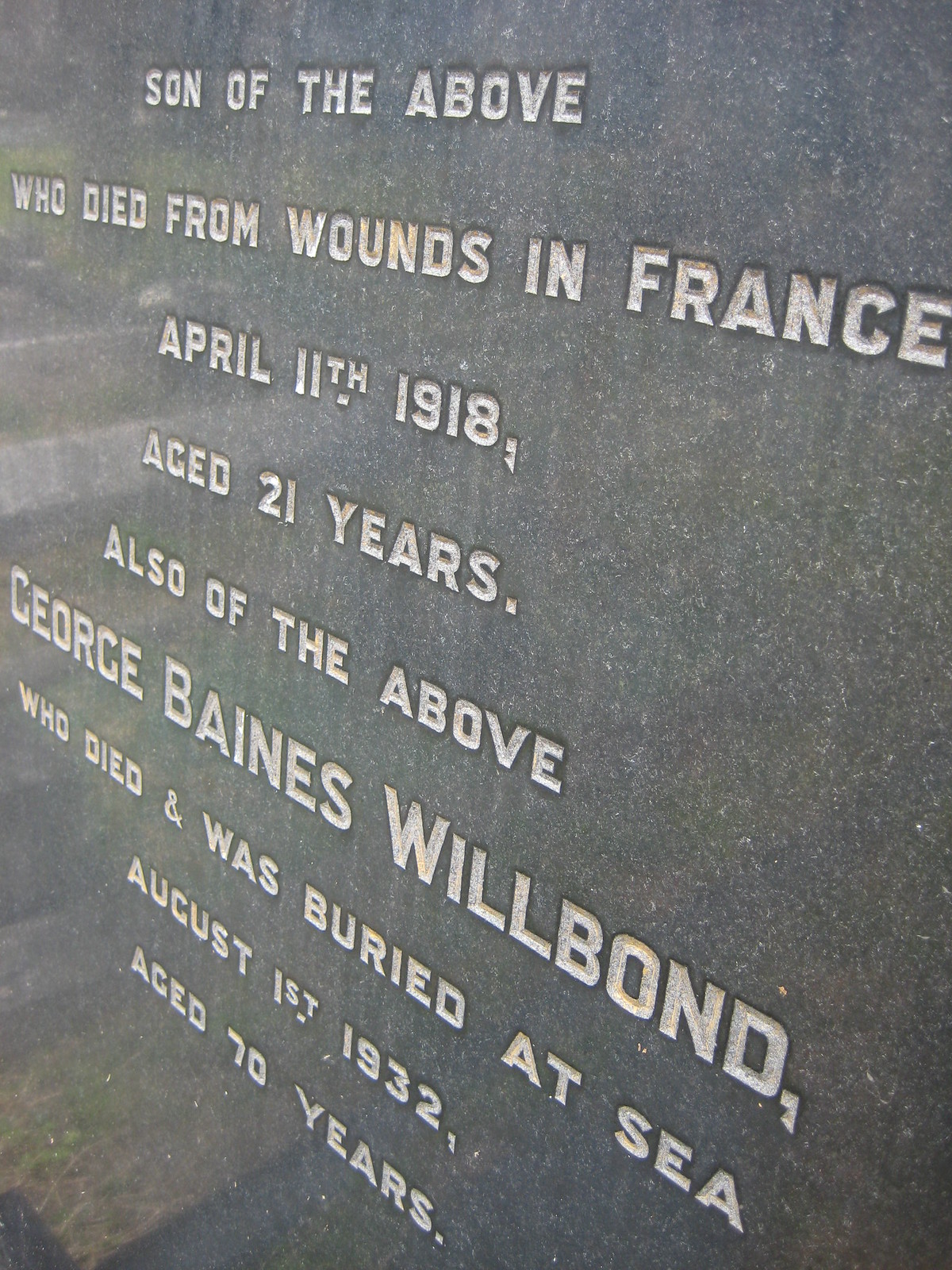The image features a gray, speckled stone plaque serving as a memorial, with no visible border. The monochrome plaque has deeply engraved, capitalized white text, central to the stone’s surface. The inscription details the memorialization of two individuals: "Son of the Above, who died from wounds in France, April 11th, 1918, aged 21 years. Also of the Above, George Baines Wilbond, who died and was buried at sea, August 1st, 1932, aged 70 years." The tribute bears a solemn, granite-like appearance, reminiscent of a tombstone, paying homage to historical figures, including a war hero who succumbed to injuries from the war.